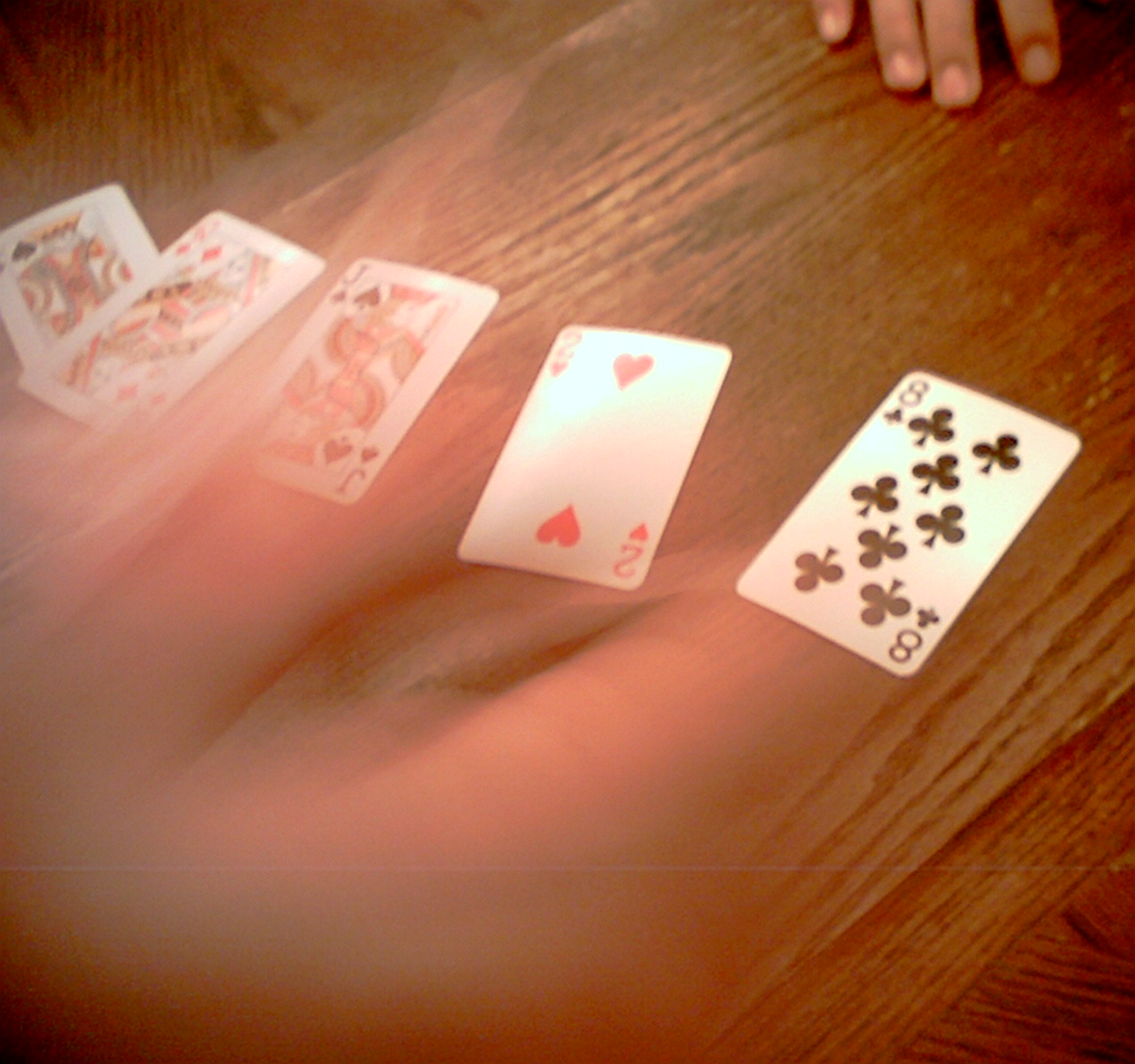This photograph captures a moment of someone playing cards on a maple-colored, wood-grained table that fills the entire frame. In the top right corner, the four fingers of a person's right hand, from the top knuckles down, rest on the table. At the center of the image lie five playing cards: an eight of clubs on the far right, a two of hearts next to it, followed by a jack of spades, a queen of diamonds, and a king of either clubs or spades, though it's not entirely clear. The foreground of the picture appears slightly out of focus, possibly due to the camera shaking during the shot, adding a soft blur to the scene.